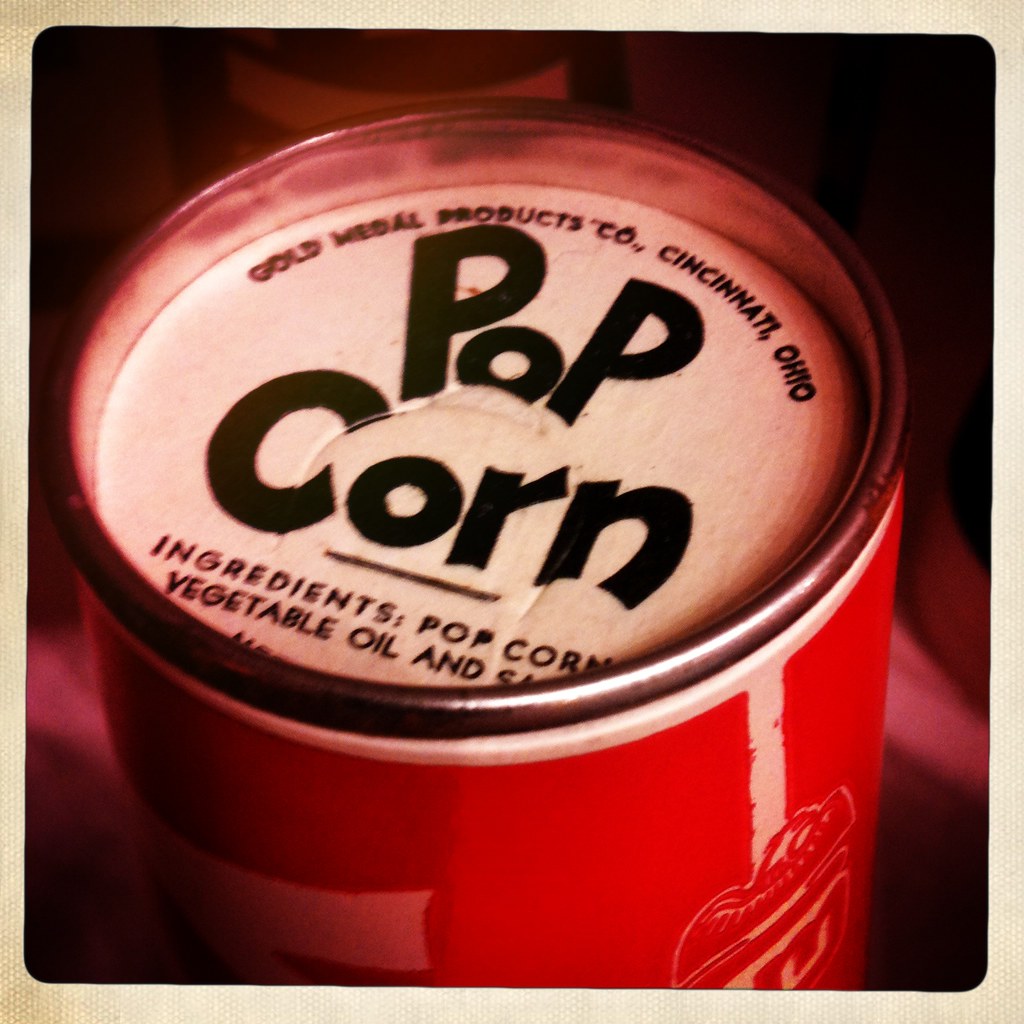This detailed image showcases a close-up of an old-style can, displaying characteristics typical of 1960s-era packaging. The can, which has a thick metal build, is adorned with a red label and a metal rim around the top. The partially inset lid prominently features the text "Popcorn" in black bold letters, with an eye-catching typography where the letters "P" are uppercase and the "o" in "Pop" is lowercase, while "Corn" follows with a similar pattern. Above the word “Popcorn," arching around the circular lid, it reads "Gold Medal Products Company, Cincinnati, Ohio." Below "Popcorn," the ingredients are listed: "Popcorn, vegetable oil, and salt," although the word "salt" is partially cut off and not fully visible. The photograph, although slightly blurry due to low lighting and possibly a shaky camera, captures the intricate details of the can’s design and label. The border surrounding the image resembles a beige Polaroid frame, adding to the vintage feel of the presentation. This nostalgic item, likely dating back to the 60s, seems to be a pre-canned popcorn product, complete with vegetable oil and seasonings, reminiscent of an era before microwave popcorn became commonplace.